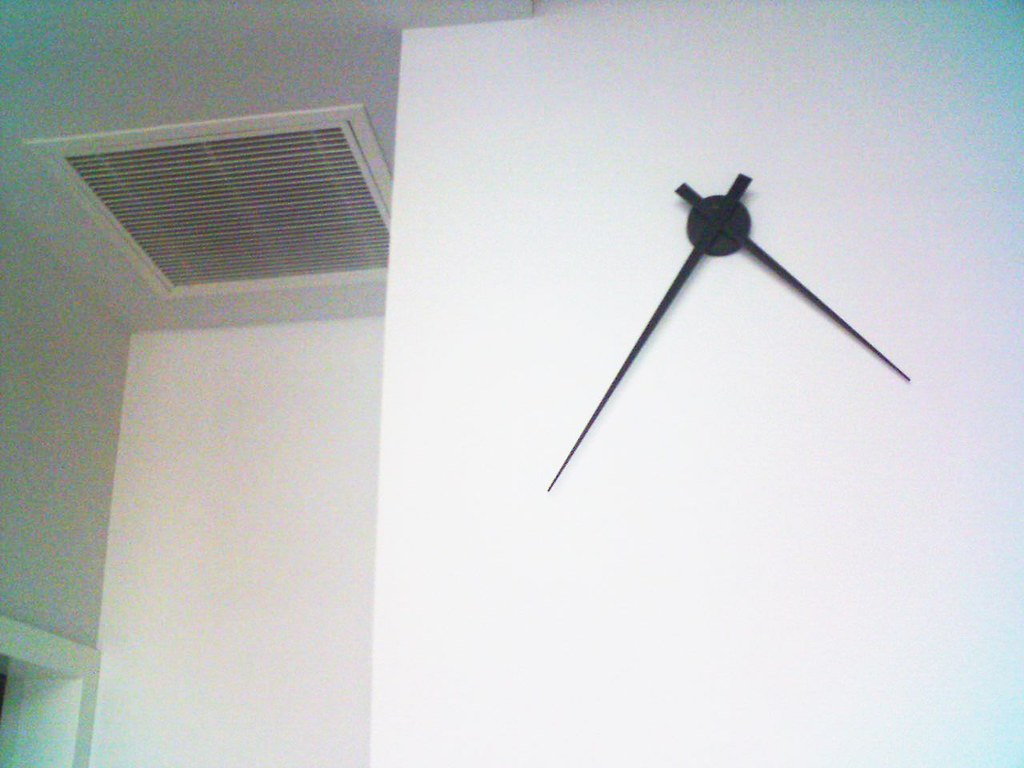A meticulously monochromatic room features a strikingly minimalist design, dominated by shades of pristine white. On the right-hand wall, illuminated under soft lighting, is an atypical clock face displaying only minimalist hands without any numerical markers or time symbols, leaving the exact time to the viewer's interpretation. This section of the wall juts out, creating a recessed area adjacent to it. Within this recess on the ceiling, there's a sizable grill—a likely component of the ventilation system. On the left side of the image, the edge of a doorway can be seen, suggesting an exit from this starkly designed space. The room's simplicity and minimalist aesthetic draw attention to these unique architectural details.